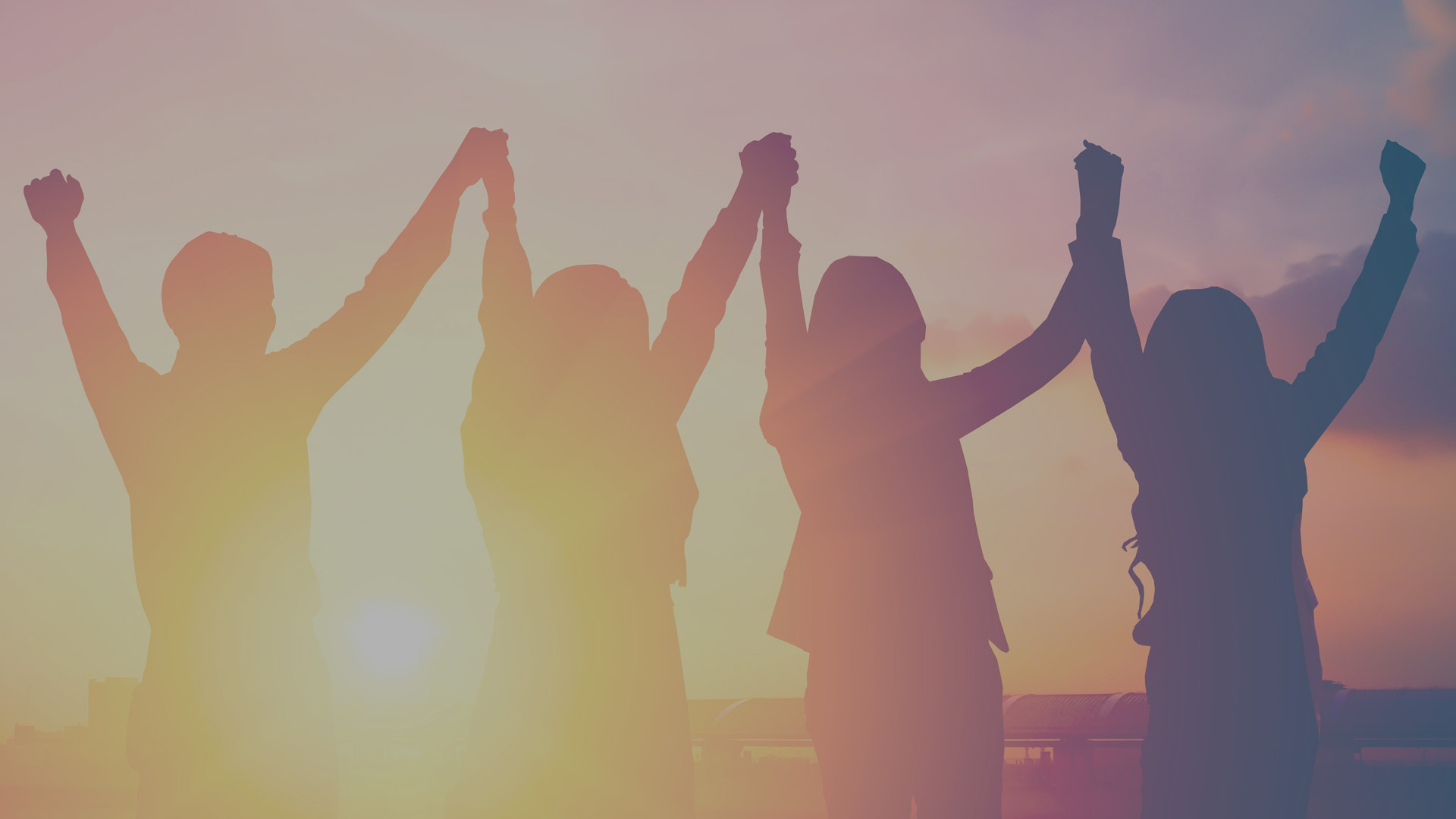The image is a color photograph in landscape orientation, capturing a vivid, picturesque moment. The photo features four individuals standing side-by-side with their hands raised triumphantly above their heads, holding each other's hands in a display of unity and victory. The group comprises one man on the far left and three women to his right. Their silhouettes, rendered in dark purple to black, stand out against the soft gradient of the sky, which transitions from lavender at the top to a warm orange near the horizon. The sun, positioned between the man and the first woman, appears bright and almost white, casting a radiant glow. To the right of the sun, a path leads towards a body of water, adding depth to the serene backdrop. The overall composition exudes a sense of camaraderie and triumph, with the raised hands spanning the entire width of the image. The photograph embodies elements of representationalism and realism, with a slightly hazy atmosphere enhancing its dreamlike quality.